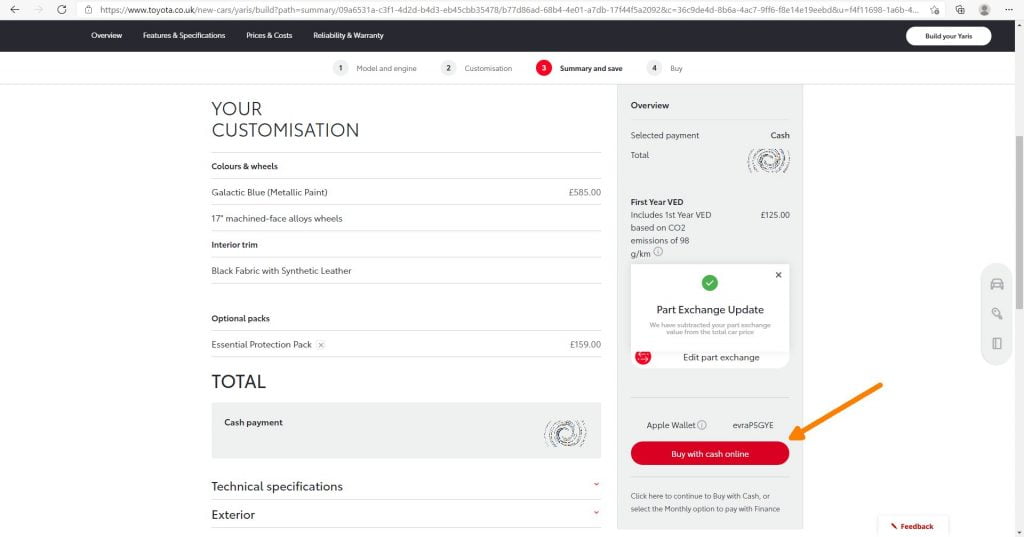This screenshot showcases an overview of features and subscriptions for a customizable product. The details, while small in font, provide comprehensive information. Featured elements include pricing and costs, the year of customization, and options for exterior colors and wheels. Additionally, there are two interior trim options—black fabric with synthetic leather. Optional packages, like the Essential Protection Pack priced at $159, are also visible.

The screenshot also outlines technical specifications and provides details on total cash payment options. The selected payment method section shows a white square and a black "Part Exchange Update" option, with editable settings. There is a red rectangle indicating the choice to "Buy with Cash Online."